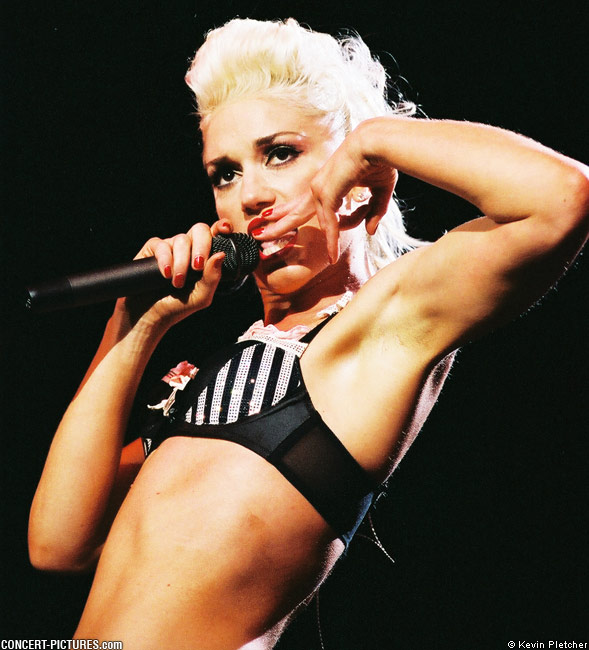In this dynamic photograph of Gwen Stefani performing on stage, she is captured from the waist up, filling almost the entire frame. Gwen, with her striking platinum blonde hair styled up at the back, is leaning slightly backward, creating a diagonal line with her body. She holds a wireless microphone close to her mouth with her right hand, while her left arm is bent, fingers pointing towards her face, adorned with bright red fingernails. Gwen's expressive dark eyes, eyelashes, and eyebrows stand out against the bright stage spotlight shining down from above, illuminating her distinctive red lipstick. She wears a short, cropped black and white striped top, which glitters with what appears to be tiny rhinestones. The background is stark black, providing a dramatic contrast that accentuates her presence. At the bottom left corner, the image credits "concert-pictures.com," while the bottom right reads "Kevin Pletcher."